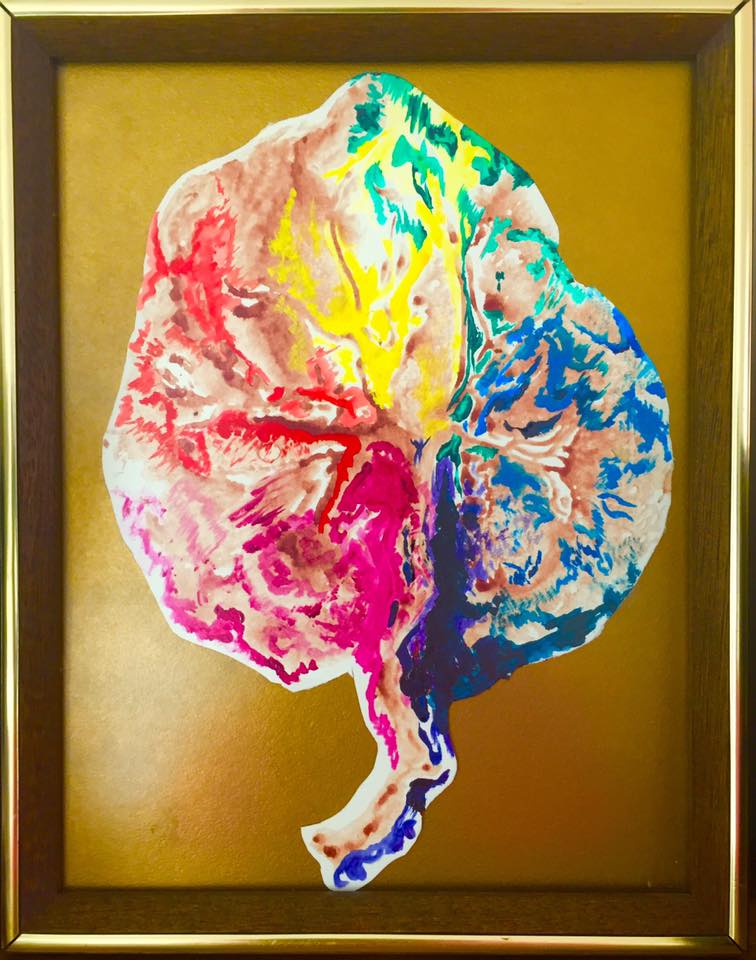The art piece is a vibrant and intricate abstract painting, encased in a wooden frame adorned with gold edging, set against a golden brown matte background. Dominating the center of the frame is a large, brain-like shape that almost touches the edges of the frame. This shape, though not a leaf, suggests organic or sculptural qualities with ridges, valleys, and a stem-like structure at the bottom. The painting is awash with a rich palette of colors, featuring hot pink, dark red, light pink, bright yellow, turquoise, royal blue, navy, medium blue, and burnt orange. The colors flow together, reminiscent of watercolor, creating a dynamic and cohesive composition. The upper left quadrant is primarily yellow, transitioning to red and pink in the lower left. Green and blue mix in the upper right, darkening into purple in the lower right. This multi-colored form, filled with crevices and craters, provides a striking contrast against the golden brown background, making it a centerpiece within the gilded frame.